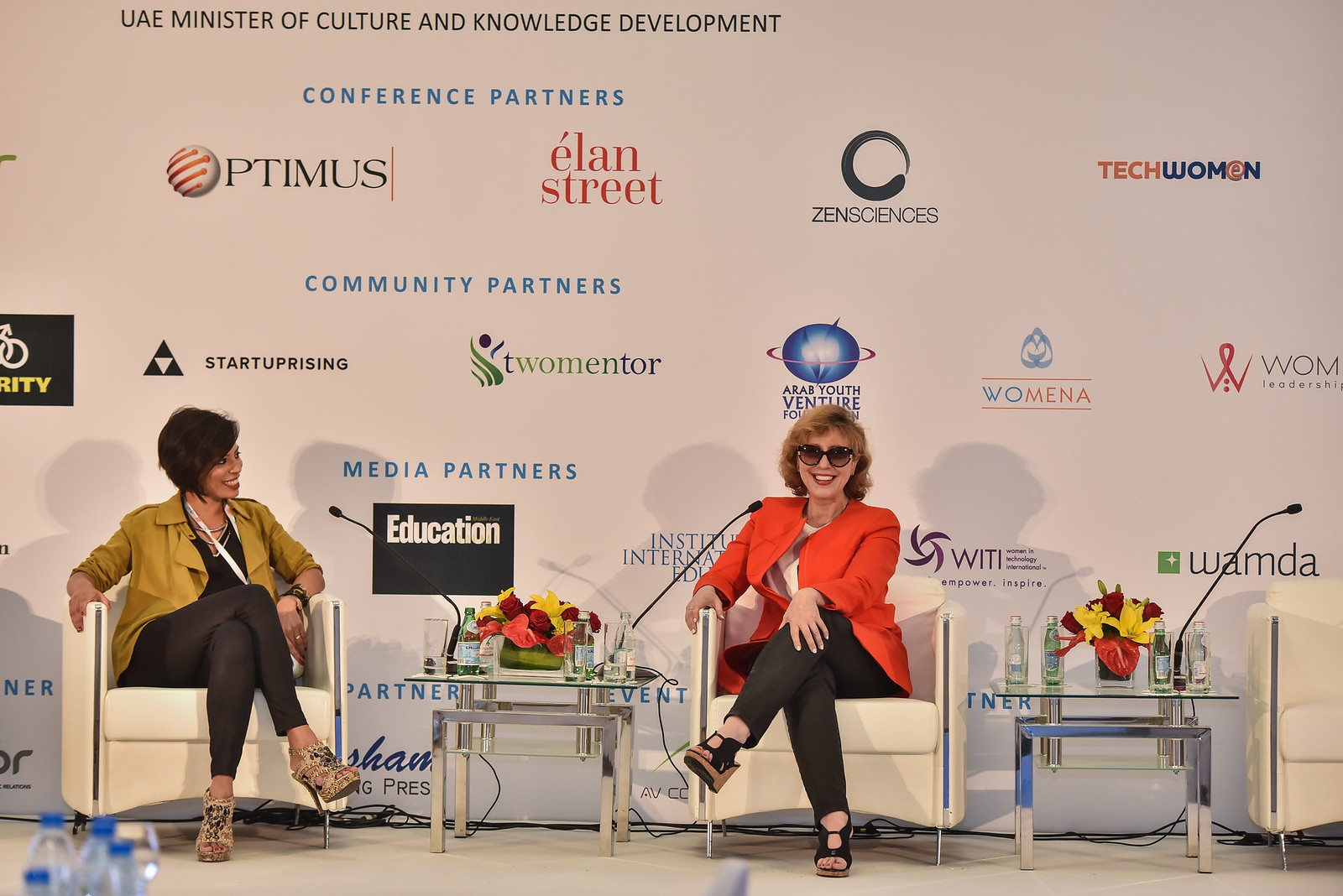The rectangular photograph depicts a conference stage with two women seated in white chairs and a third empty chair to the far right. The backdrop is adorned with numerous logos from various sponsors, including Optimus, Elon Street, Zen Sciences, Tech Woman, Start Uprising, 2Mentor, Wamena, Education, WITI, and WAMDA. At the top of the backdrop, it reads "Conference Partners" and features a header noting involvement from the UAE Minister of Culture and Knowledge Development.

The woman on the left has dark brown hair and is wearing a gold top over a black shirt, black leggings, and high-heeled shoes. She smiles while looking at the other woman, who has dirty blonde hair, is wearing sunglasses, and dressed in an orange blazer over a white shirt, with black leggings and sandals. Microphones are extended towards both speakers.

Between the women are chrome-based tables with glass tops, holding vases of fresh flowers, various beverages, and glasses. The nearest corner of the image shows the tops of clear water bottles with blue caps. The woman in the orange jacket is facing the camera with her legs crossed, while the woman in the gold top directs her smile towards her.